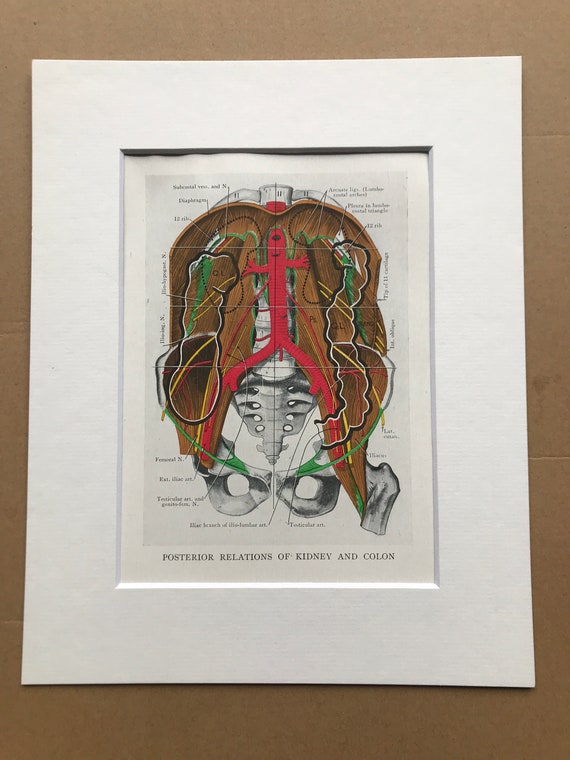This is an image of a vintage medical illustration hanging on a medium brown wall. The thick white frame surrounds the detailed diagram, giving it a distinguished presentation. The illustration, set against a white background, appears to be an old anatomical chart titled "Posterior Relations of Kidney and Colon" at the bottom. It meticulously depicts the anatomical connections between the kidney and colon. Brown-colored muscles, red veins, and highlighted regions in black, white, and green outlines dominate the visual. Yellow lines trace various anatomical pathways, while black lettering provides annotations, though the text is hard to decipher from the photograph's distant perspective.